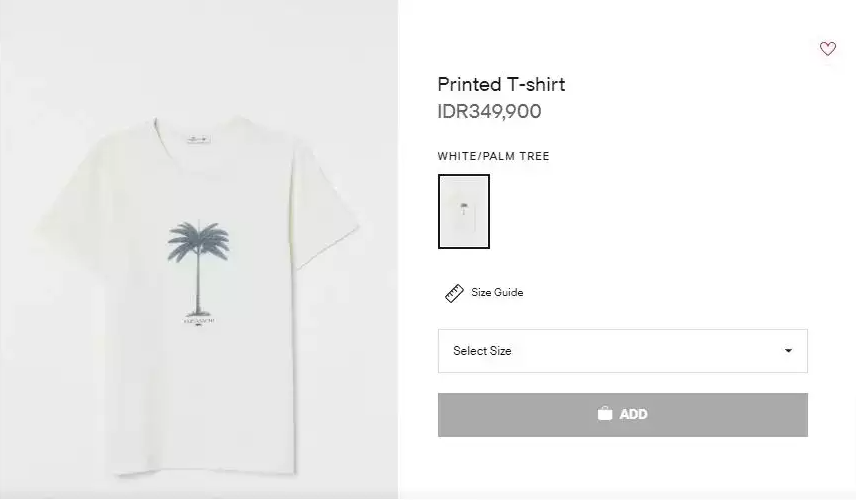This image is a screenshot from an unidentified e-commerce shopping site displaying a product page with a monochromatic color scheme. The left half of the page is shaded in light gray and showcases a white t-shirt adorned with a palm tree graphic. The depiction of the palm tree appears washed out, leaving it unclear whether it is in black and white or in color. 

On the right half, which is solid white, detailed information about the shirt is provided in black text. The shirt is labeled as a "Printed T-Shirt," priced at IDR 349,900. The currency IDR suggests it is measured in Indonesian Rupiah. Below the price, the description "White / Palm Tree" is displayed, accompanied by a small thumbnail image of the shirt mirroring the main image on the left. There is a ruler icon labeled "Size Guide" for additional sizing information. 

Beneath these details, there's a drop-down bar for selecting the shirt size and a gray button featuring a handbag icon that prompts "Add" for adding the item to the shopping cart.